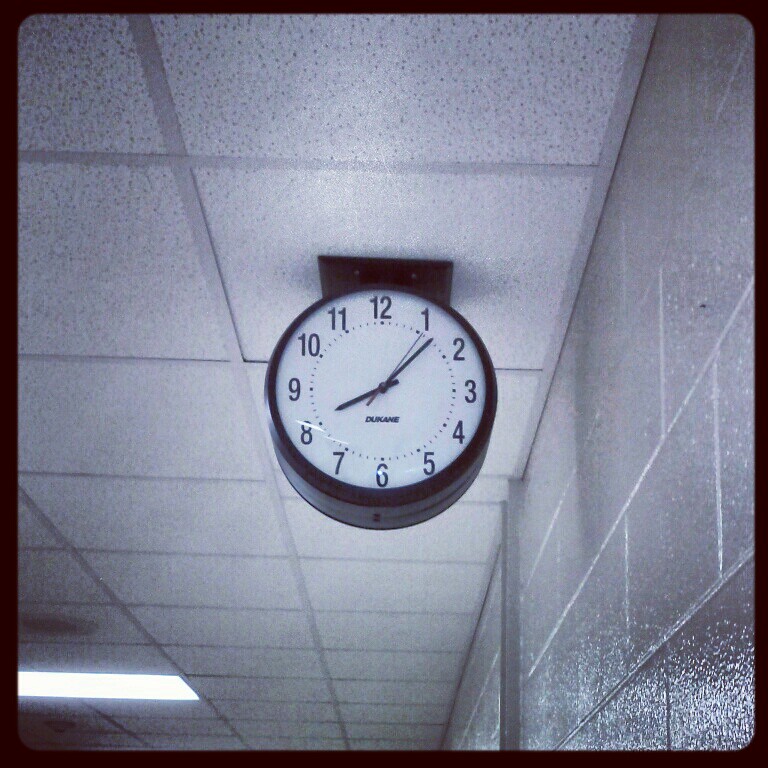This photograph is bordered with a brown frame, complementing its monochromatic theme. The image mainly features black, white, and gray tones. The ceiling is a drop-down style commonly found in office buildings, with removable panels. Each tile is white, speckled with gray, and has visible bands running across them. Hanging from the center of the ceiling is a vintage clock with an analog face. The clock displays the time as 8:07 and 5 seconds, with black numbers from 1 to 12 and traditional hour, minute, and second hands. The clock is supported by a metal fixture attached to the ceiling. To the right of the image, shiny cement walls with noticeable grout lines are visible, suggesting the setting might be an office building or a school hallway.